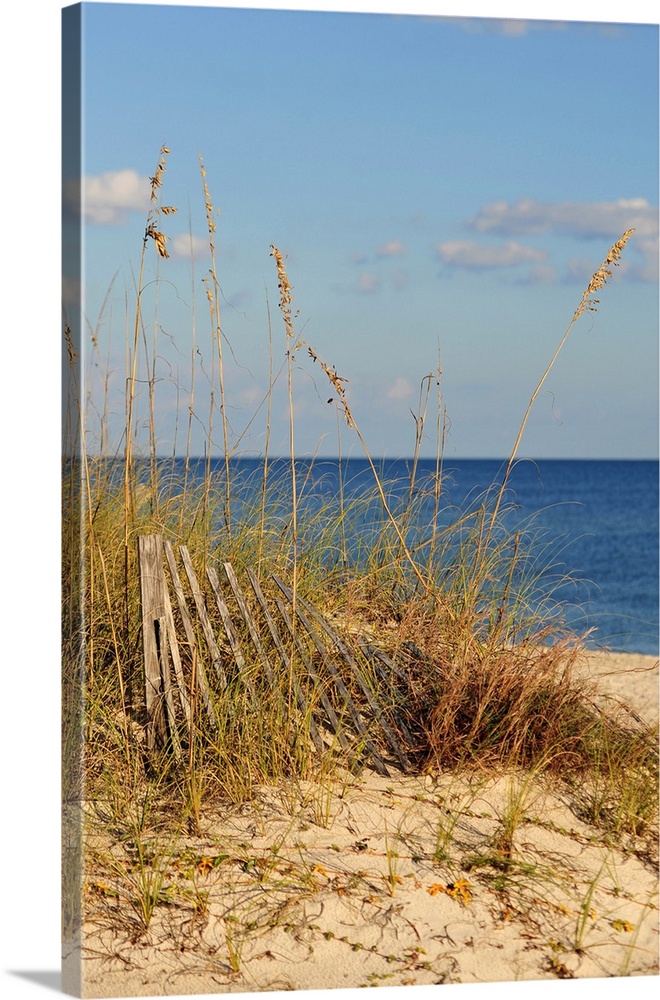The image depicts a three-dimensional canvas standing vertically against a white backdrop, casting a subtle shadow behind it. The artwork on the canvas illustrates a serene beach scene, featuring a tranquil dark blue ocean beneath a sky adorned with distant clouds. The foreground displays a stretch of beige sandy beach, accented by patches of weeds and brush positioned close to the photographer. Adding to the scene's charm, a faded wooden fence with vertical slats, partially collapsed, mingles with the surrounding brush, enhancing the rustic ambiance of the beach landscape.